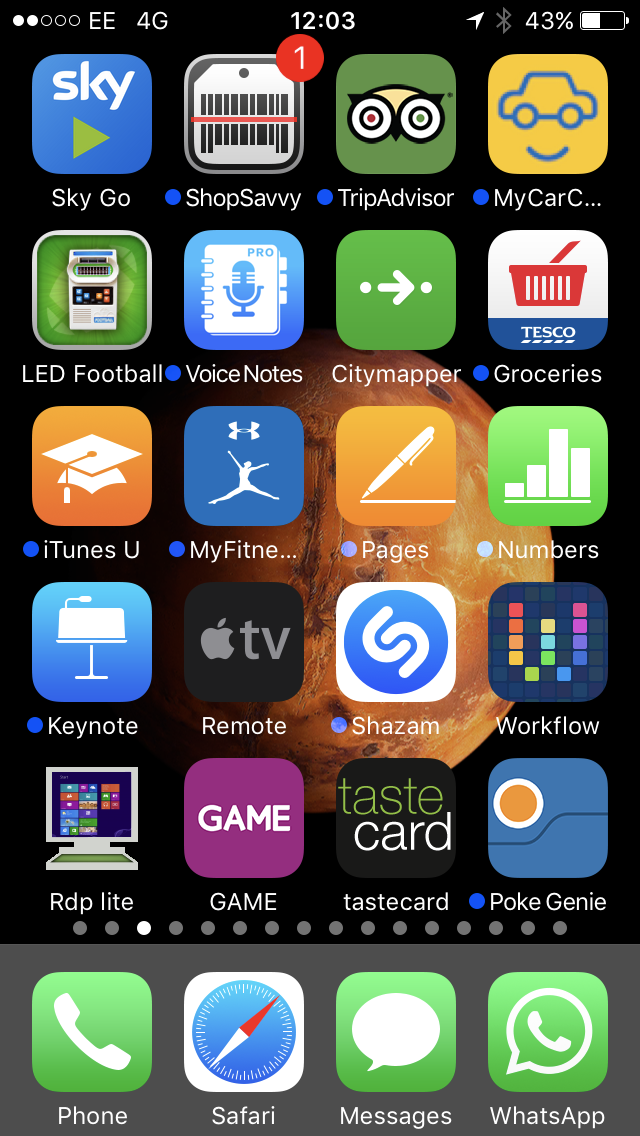The image displays a smartphone home screen with various app icons arranged on a black background. The device is connected to a 4G network and showcases the time as 12:03 PM. The battery level is at 43%. The app icons are neatly organized in a left-to-right and top-to-bottom sequence. The first row features Sky Go, Shop Survey, and Trip Advisor. The second row comprises My Car, LED Football, and Voice Notes. Following in the third row are City Mapper, Tesco Groceries, and iTunes. The fourth row consists of My Fitness, Pages, and Numbers. On the fifth row, we see Keynote, Remote TV, and Shazam. The sixth row includes Workflow, RDP File, and Game. Finally, the bottom row has Taste Card and Poke Genie. Each app icon is distinct in color, creating a vivid mosaic against the dark background.